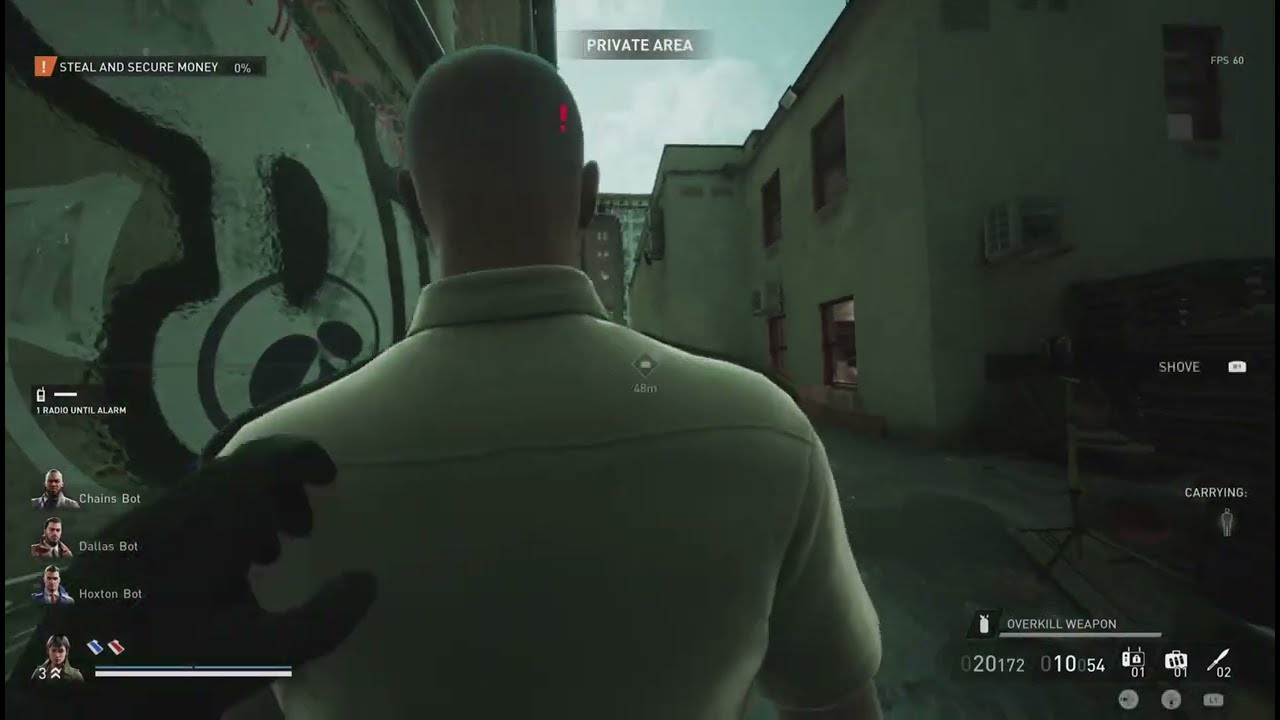In this dark and moody combat video game image, the player's perspective is a first-person view, with their left hand reaching out, as if about to tap or grab a bald man with a very short haircut and a light green collared shirt. The man stands in the center facing away, within a narrow alley flanked by old concrete or adobe buildings. Prominent graffiti, including a skull design, adorns the wall to the left. The setting is outdoors under a clouded sky, suggesting twilight. The user interface displays various game elements such as mission objectives ("steal and secure money"), player choices including "Haim Chains Bot, Dallas Bot, Hoxton Bot," weapon options, and action prompts like "shove" with the R1 button. At the top of the screen, it indicates "private area," further immersing players in the atmospheric world of this intense shooter game.